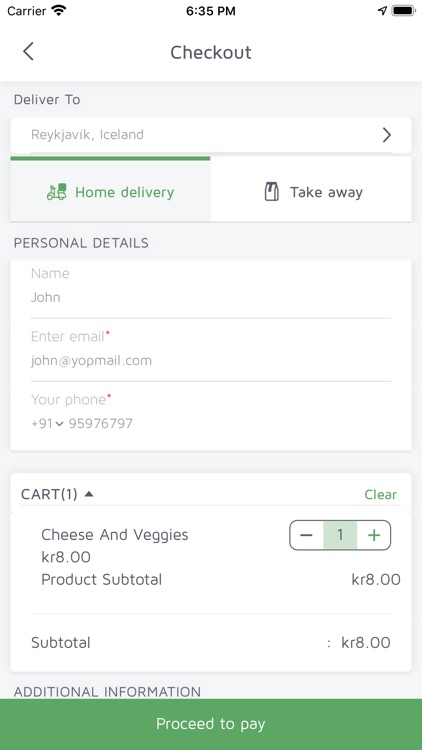The image depicts a user interface of a delivery app where an individual is in the process of filling out delivery details. The screen shows that the delivery destination is Reykjavik, Iceland. The personal details section is populated with placeholder information, including the name "John," an email address "john@yapmail.com," and a phone number. The delivery method selected is home delivery. The shopping cart contains only cheese and vegetables, with the total cost amounting to 8.00 KR (likely Icelandic Krona). The app's interface features a predominantly white and gray color scheme with green accents. A "Back" button is visible, as well as a "Proceed to Pay" button at the bottom of the screen. Additional phone details visible in the image show a full battery, active location services, and a strong Wi-Fi connection.